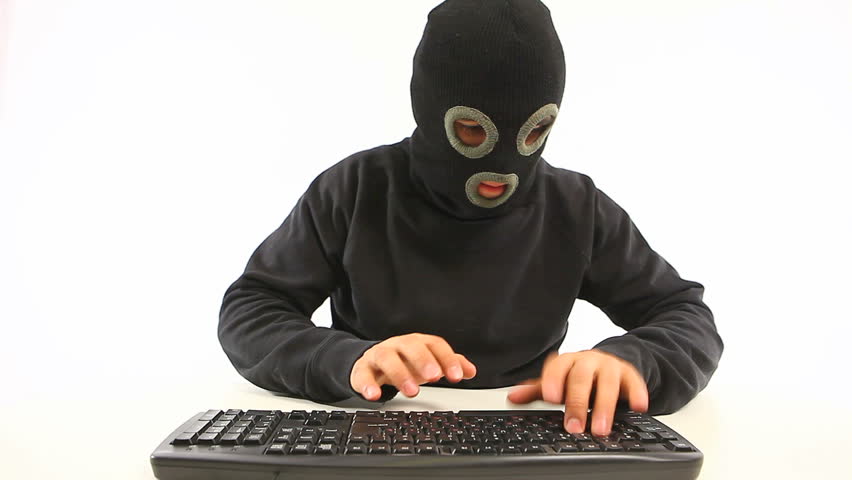This color photograph, potentially AI-generated, features a man against a completely white, blotted-out background. The man is wearing a gray ski mask with lighter gray outlines accentuating the eye and mouth cutouts. His eyes, which are directed downward, and his lips, which appear somewhat unnatural, suggest the possibility of digital manipulation. He is dressed in a long-sleeve gray shirt and is seated at a gray keyboard. The image raises further suspicion due to the peculiar appearance of his hands: his left hand’s middle and ring fingers seem normal, while the index and pinky fingers are visibly truncated, missing the last two joints. Conversely, his right hand appears disproportionately large. These anomalies, particularly the unnatural look of the lips and the distorted fingers, strongly suggest that this might be an AI-generated image, and not a flawless one at that.